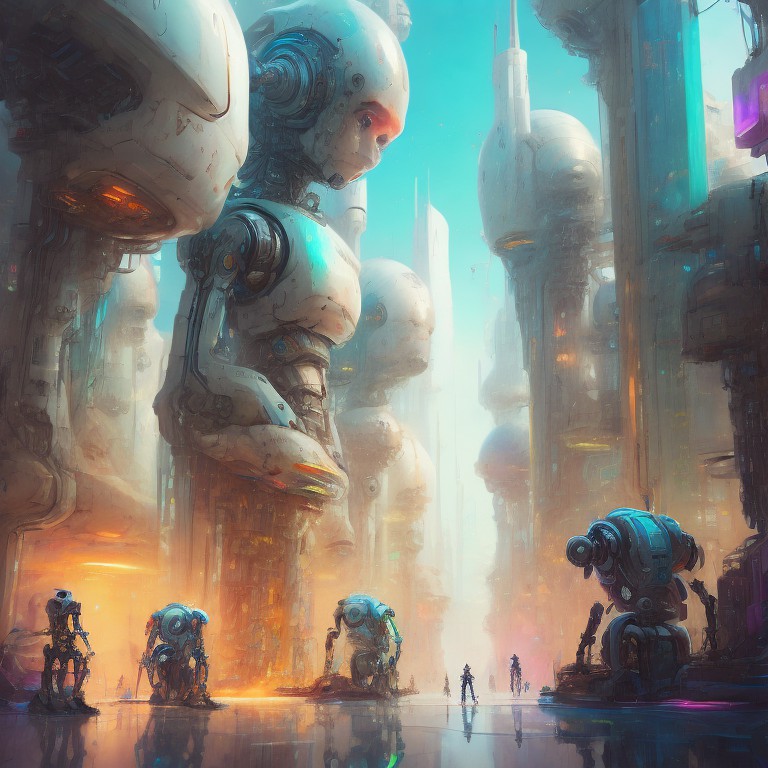The image is a detailed, fantasy futuristic painting featuring a variety of robot-like figures. Dominating the scene are several large robots resembling astronauts with round helmets, white chest plates, and silver lower bodies, arms, and ears. Their heads are bent down, seemingly observing the ground. The robots' white heads have red, eyebrow-like markings, and their mechanical bodies are highlighted against a light turquoise sky. In the background, tall vertical buildings create an urban landscape.

Below these large robots are smaller versions, some appearing as tiny as fighters, moving about on a slick, glass-like surface. These smaller robots vary in size and are depicted with some humanoid features, walking on human-like legs. The ground surface includes a small green strip at the bottom and patches of yellow and violet illuminations, adding a vibrant touch to the otherwise muted color palette of the scene.

The central large robot, evoking a baby-like appearance, stands out prominently, flanked by another tall structure that appears to be a fish with a tower on its head, and another more abstract, less human-like robot. The composition on the surface reflects an organized yet fantastical hierarchy, with the smaller robots potentially acting as subordinates to their larger counterparts. The overall color scheme is hazy but includes shades of sky blue, salmon, yellow, and tan, adding to the painting's surreal and imaginative atmosphere.